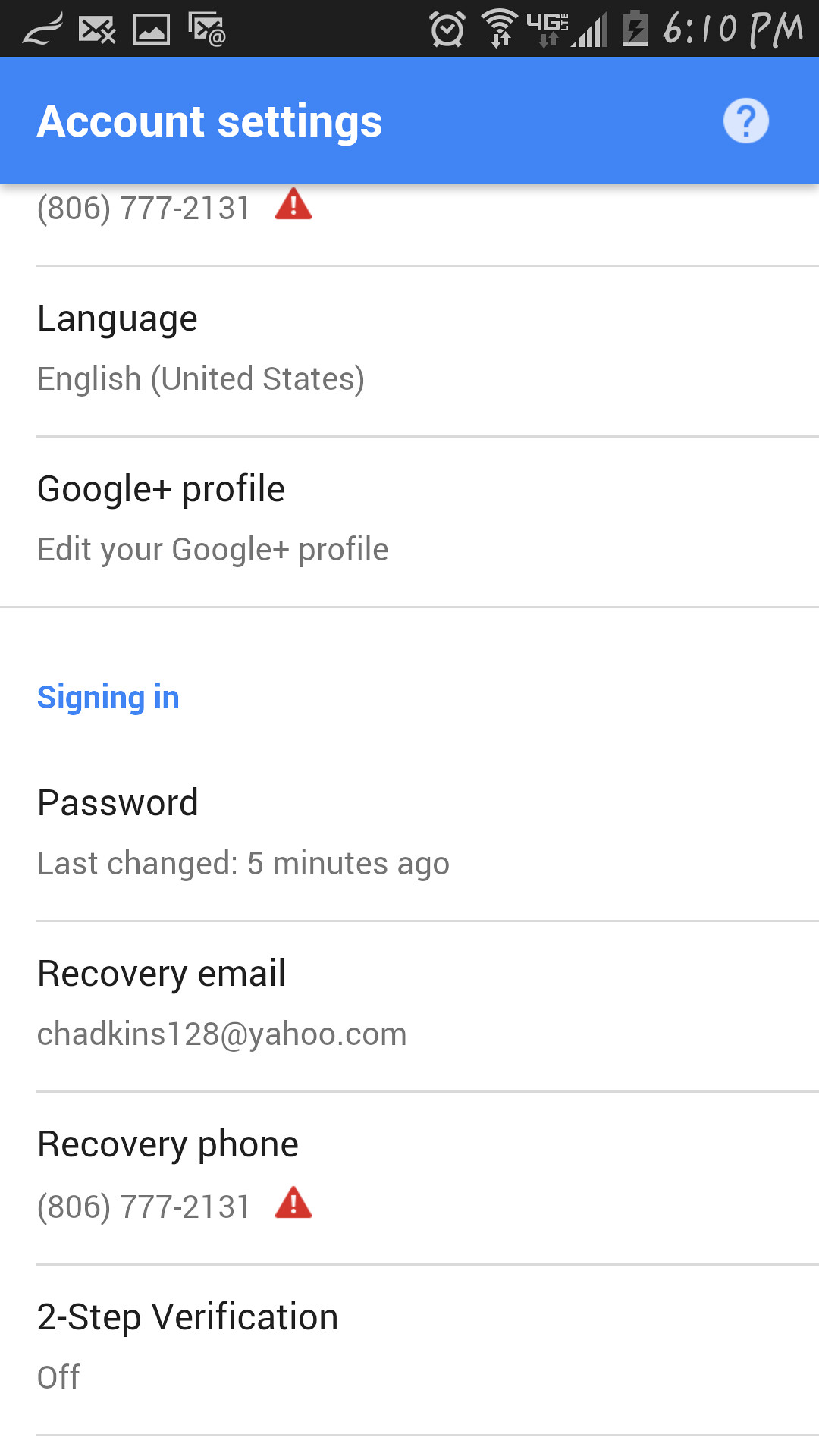**Detailed Caption:**

This image is a screenshot of a phone displaying a user’s settings profile. The screen is organized in a vertical format, likely indicative of a smartphone interface—possibly an Android device, although the exact type is not confirmed.

At the very top of the screen, there's a black status bar containing essential device information, including the time, displayed as 6:10 PM. The status bar also shows a low battery indicator, four signal bars, a 4G network connection, and a strong Wi-Fi signal.

Directly below the status bar, there's a prominent blue bar with the label "Account Settings". This title is repeated just below the blue bar in a larger font on a white background. The profile section underneath begins with a phone number: "806-777-2131", accompanied by a warning icon which suggests some notification or issue related to this number. The phone number is labeled as an English (United States) contact.

Further down, there's a section for Google Plus profile management, marked by the text "Edit your Google Plus profile."

The next segment details the security and recovery options:
- The section starts with "Signing in" information, stating that the password was changed 5 minutes ago.
- It includes a recovery email address: Chadkins128@yahoo.com.
- The recovery phone number is repeated as 806-777-2131.
- Additionally, it's noted that two-step verification is currently turned off.

The overall layout, from the status bar to the security options, reflects a standard mobile interface captured in a screenshot, likely for personal reference or technical troubleshooting.